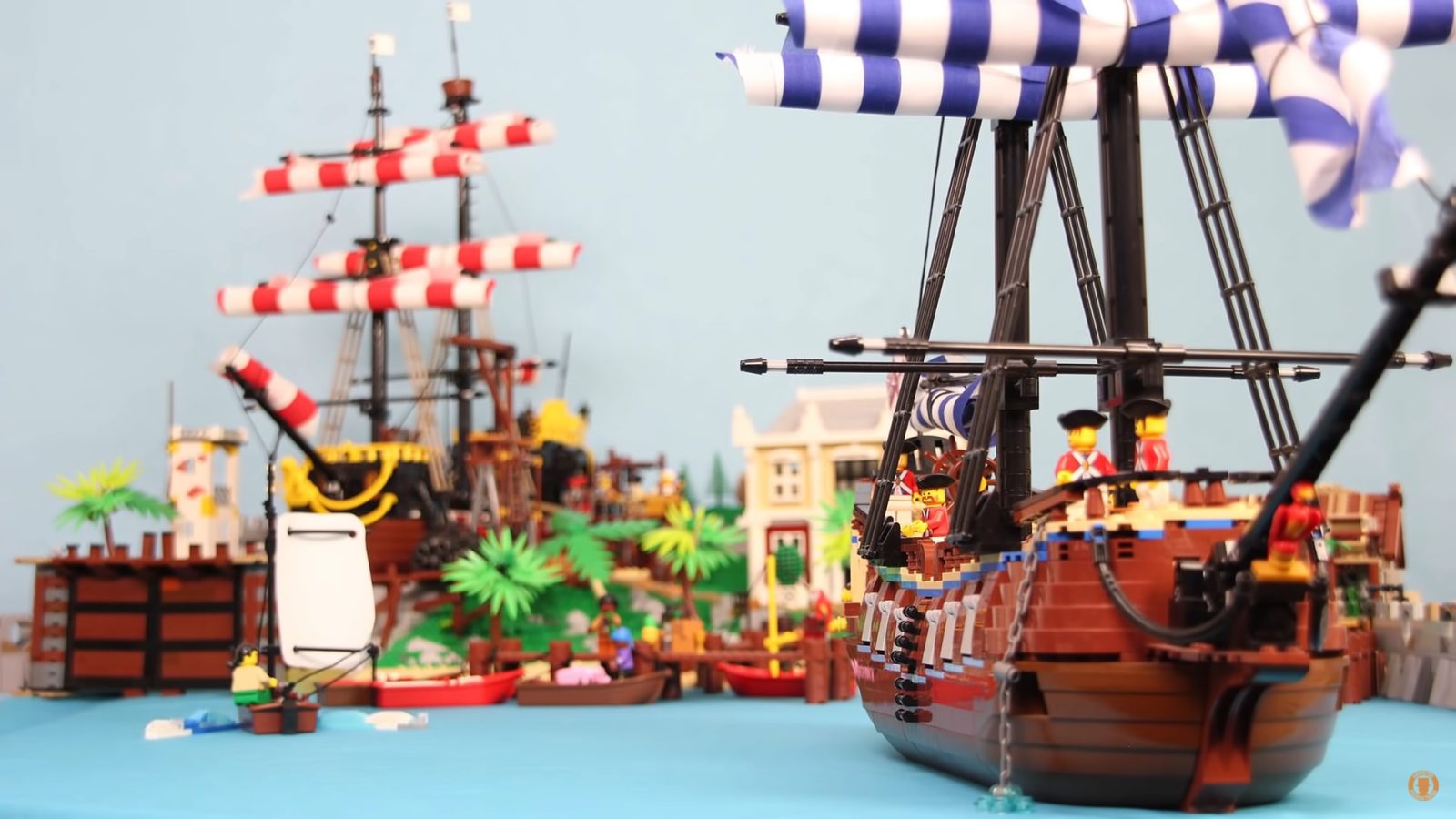The image showcases an intricately detailed Lego set, primarily focused on a colonial maritime scene. At the forefront on the right side is a Lego ship adorned with blue and white striped sails and a blue and white flag, manned by several Lego Imperial minifigures in red coats and black caps, some of whom are positioned nearer to the viewer while others are further back. A similar ship with red and white striped sails is visible in the background on the left. To the left of the scene, a small Lego minifigure navigates a boat with a personal sail, amidst a harbor simulated by a blue table interspersed with occasional blue Lego pieces resembling waves. The harbor is lined with a Lego dock, rowboats, and an island featuring palm trees and a yellow Lego building with a brown door and white windows. The backdrop extends into a Lego town comprised of white buildings and lush tropical vegetation, reinforcing the colonial theme and adding depth to the overall scene.